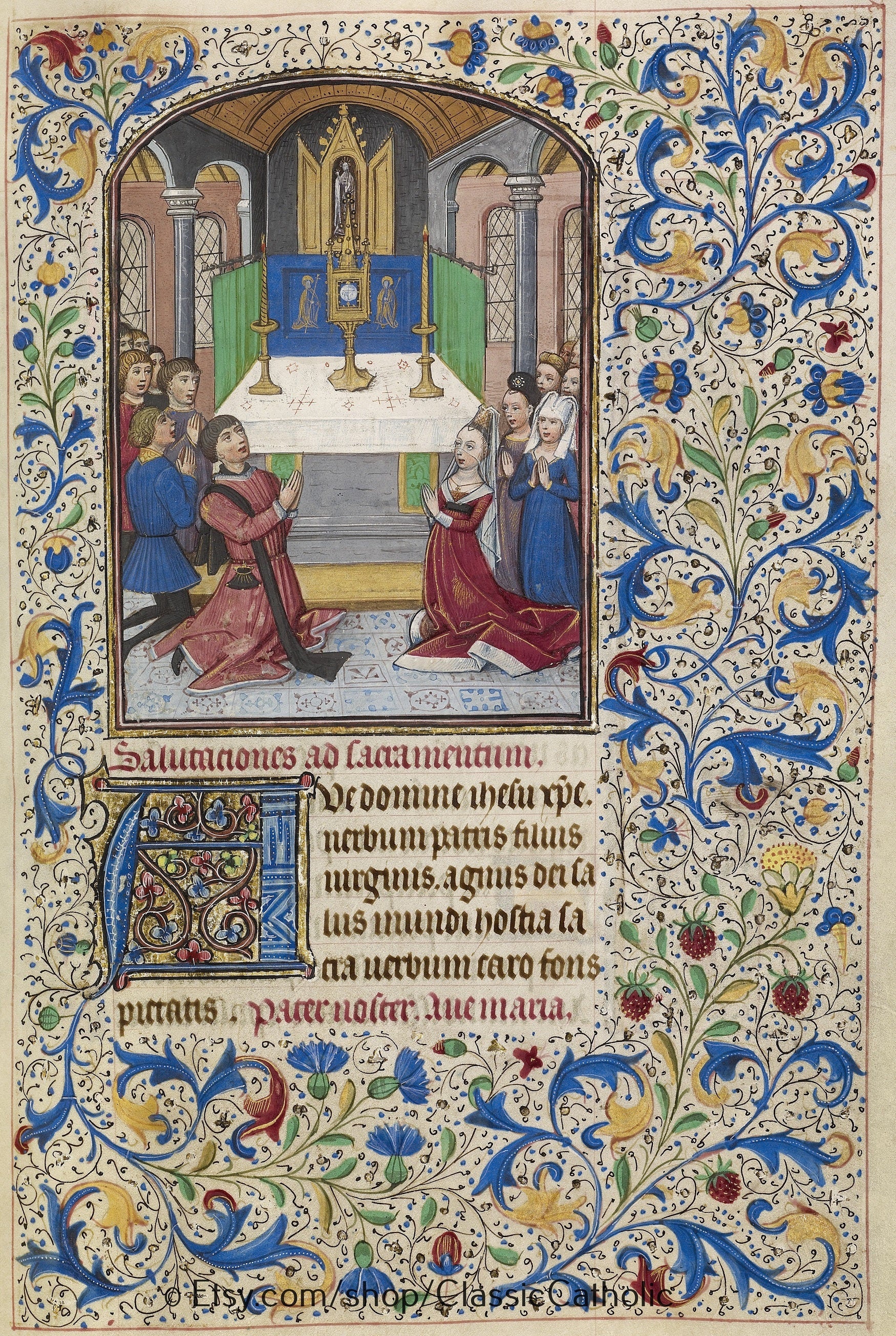This detailed image is a piece of art resembling a page from a medieval book or a poster with intricate designs. The background is an off-white shade, almost like aged parchment, and it is filled with swirling patterns and decorations in hues of blue, yellow, and green, accented with small blue spots. 

The focal point of the artwork features an image of a group of people in medieval attire, gathered around a white altar set within a church setting. The scene includes a prominent tabernacle, flanked by two tall golden candlesticks, suggesting a religious ceremony. The group, consisting of both men and women, is depicted kneeling with hands clasped in prayer.

This central image is framed by flower and petal-like designs, with notable blue petals enhancing its ornate appearance. Below this scene is a block of text written in black and light purple medieval-style script, although the specific language is not identifiable. 

At the very bottom of the page, there is a watermark indicating the source of this piece: etsy.com/shop/classicCatholic, perhaps suggesting that this elaborate, richly detailed work is intended for a market appreciative of classical Catholic art and decor.